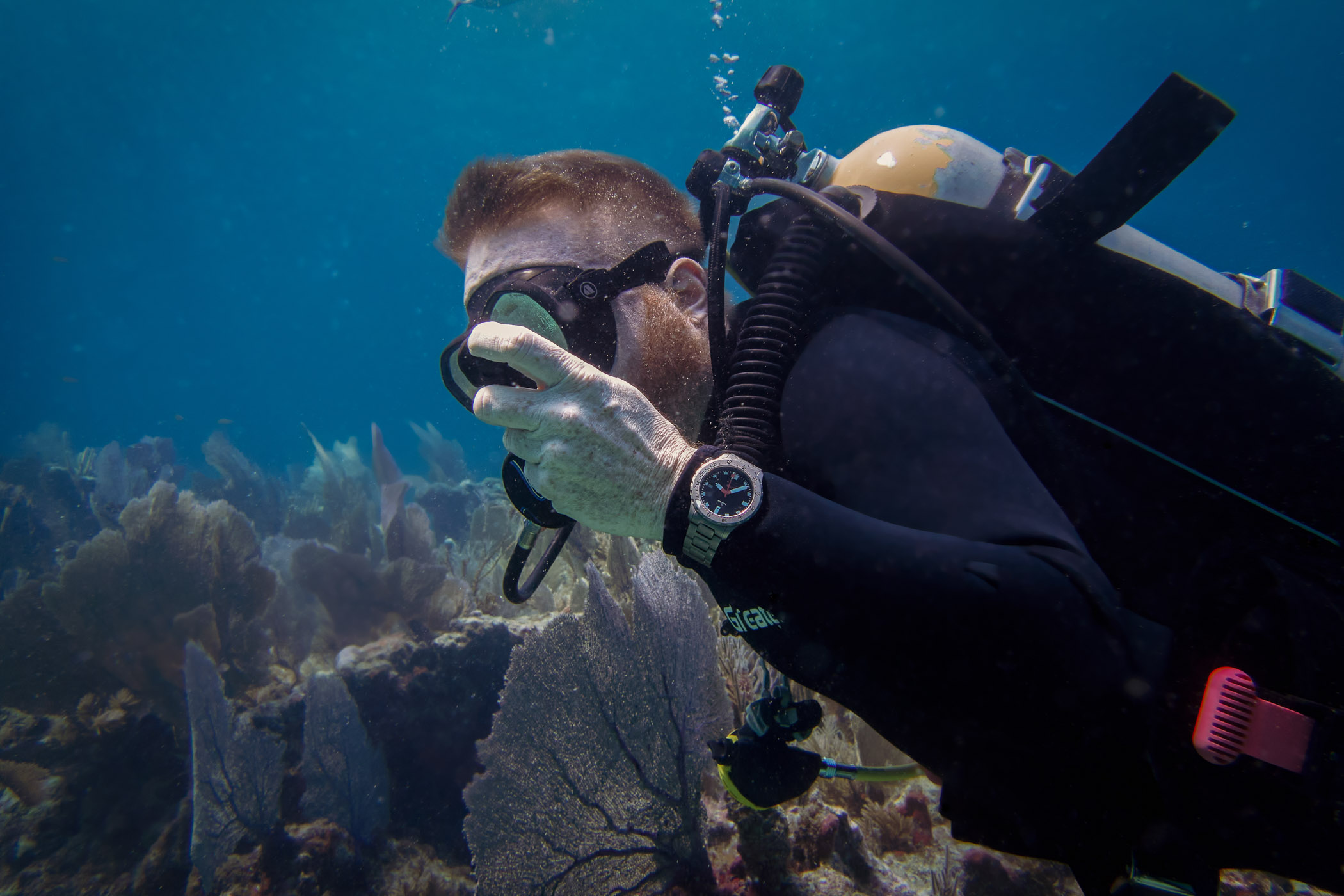The image captures a scuba diver with short, orange hair and a matching beard, exploring a vibrant coral reef underwater. He is equipped with black diving gear, including a mask connected to a regulator by a black tube, a buoyancy control device, and a tank on his back. A watch is visibly strapped over his wetsuit on his left wrist, suggesting he is monitoring his dive time. The diver has freckles on his hand, which he is holding near his mouth area. Tucked into his side is a red item, adding a hint of color to his otherwise dark gear.

The composition places the diver predominantly on the right side of the image, swimming towards the left. The background reveals a thriving underwater ecosystem with a variety of corals and marine plants, some resembling fans with dendritic patterns. The seabed is visible, showcasing different kinds of algae and other plant life. The water is clear, allowing sunlight to penetrate and illuminate the scene, creating a serene and adventurous atmosphere with no visible text. The overall impression is one of detailed exploration in a healthy, underwater world.